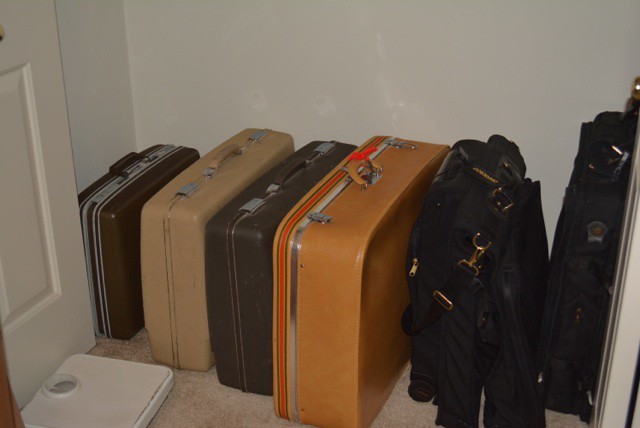This indoor photograph captures a collection of six suitcases lined up against a bare white wall, presumably in a room or closet. The suitcases are arranged in an orderly fashion, from left to right, by their size and type. Starting from the left, the first suitcase is a small, dark brown case. Next to it is a slightly larger, tan suitcase, followed by a medium-sized, brown suitcase. Adjacent to this is the largest of the hard case suitcases, a lighter brown or caramel-colored suitcase. The remaining two on the right are black, soft, shapeless suitcases adorned with gold metal pieces and straps, resembling more of a duffel or travel bag. In the foreground, near the lower left corner of the image, there is a white bathroom scale, suggesting its potential use for weighing the luggage. The floor is covered in a beige carpet, and a white door with standard rectangular indents is partially visible on the left side of the image. The suitcases, appearing worn and well-used, rest on the floor, lined up meticulously against the pristine white wall.